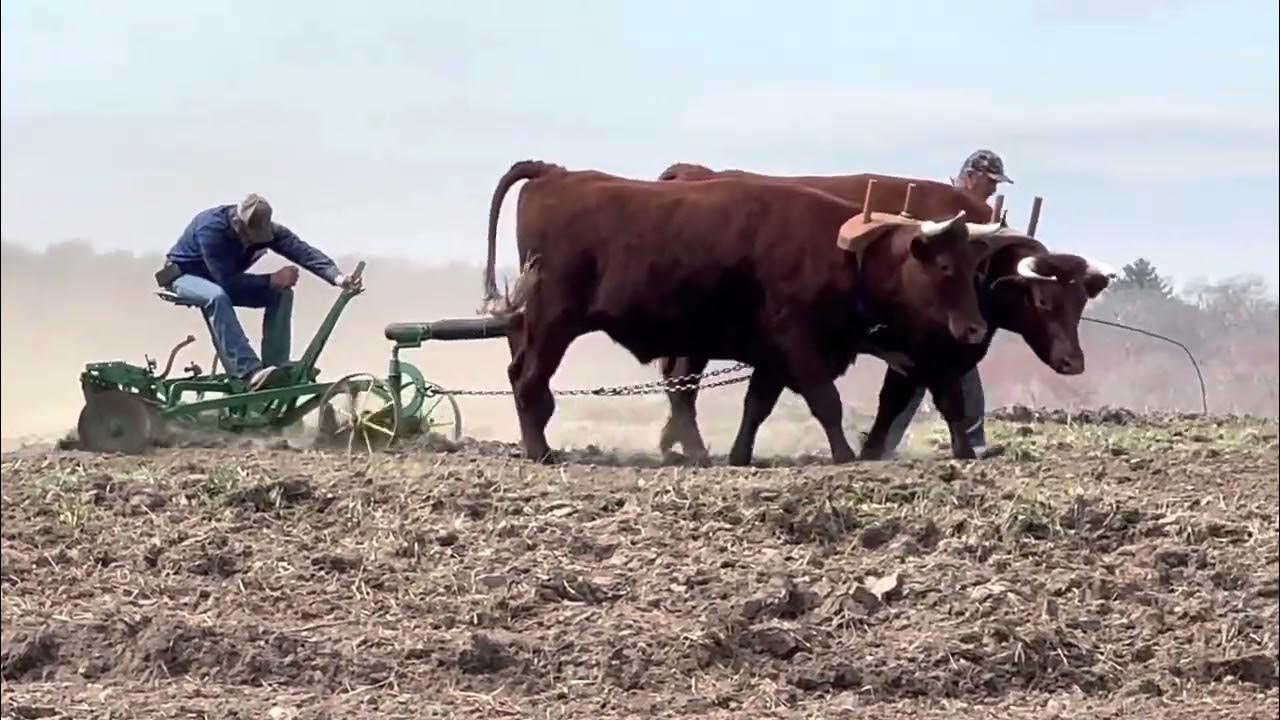In this outdoor, daytime farm scene, a pair of brown oxen with horns are diligently pulling a plow through rich, brown soil. Their heads are bowed under a sturdy yoke as they work in unison to till the land. The plow they are pulling is attached to a green mechanical vehicle, on which a man sits, operating the machinery. He is dressed in a long-sleeve blue shirt, blue jeans, and a brown baseball cap, gripping a handle as he steers. Another man, also wearing a brown cap, walks alongside the oxen, guiding them. The background features a vivid blue sky with scattered white clouds and some patches of green sprigs emerging from the soil. The entire scene captures the essence of hardworking life on a farm, emphasizing the collaboration between man and animal in agricultural labor.